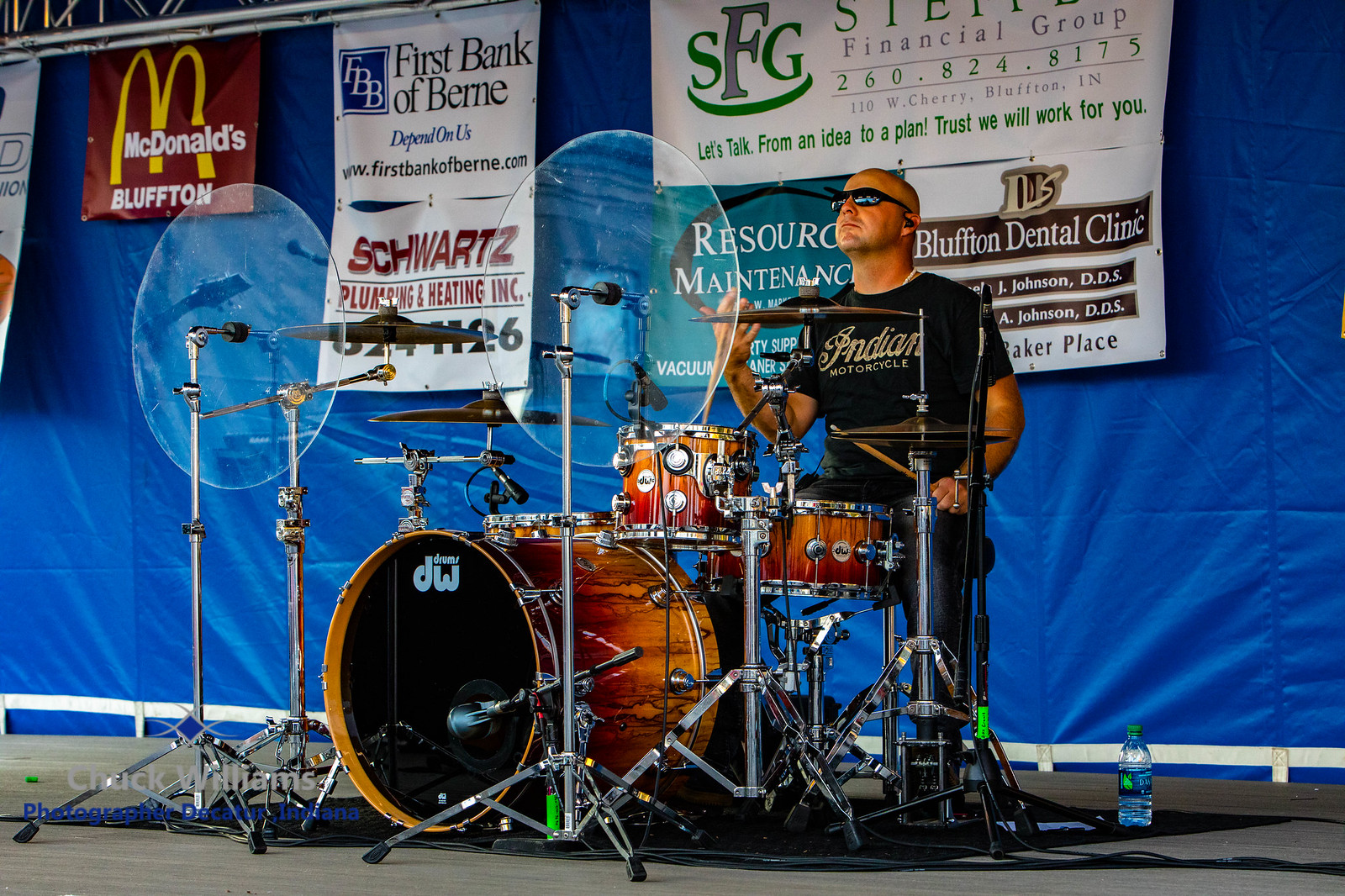The image captures a daytime outdoor music concert with a stage set against a blue backdrop. The backdrop is adorned with various banners and notices, including those for McDonald's, First Bank of Bern, SFG Financial Group, Bluffton Dental Clinic, Schwartz Plumbing and Heating, and Resource Maintenance. A drum player, wearing a black shirt with "Indian Motorcycle" written on it and blue pants, sits at a large brown drum set. He sports glasses and appears poised to play or in the midst of performing. A plastic water bottle is positioned on the lower right-hand side of the stage floor, which is grey. The photograph is credited to Chuck Williams Photography, as noted on the bottom left-hand side.